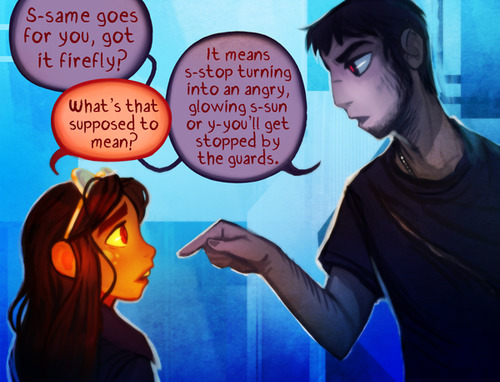This vibrant comic-style illustration features two teenagers engaged in a spirited conversation. The young man, clad in a simple black t-shirt, points emphatically at the young woman. His speech bubble reads, "It means stop turning into an angry glowing sun or you'll get stopped by the guards." The young woman, whose face is aglow with a mysterious light, retorts, "What's that supposed to mean?" Her radiant visage seems to hint at some supernatural abilities, further emphasized by the text bubble continuing, "Same goes for you, got it Firefly?" She dons glasses perched atop her head and an indistinguishable top. The scene appears set in a dimly lit, undefined background, which might be a bathroom. The interplay of dialog bubbles and the glowing effect around the girl's face adds a dynamic, fantastical quality to the image, suggesting a story rich with intrigue and special powers.